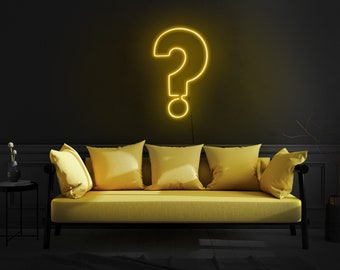The image showcases an intricately designed scene that appears to be somewhat 3D-rendered or AI-generated, highlighting its realistic yet somewhat surreal quality. At the focal point of the image is a vibrant yellow couch, illuminated softly in an otherwise dark room. The couch features five yellow, square throw pillows—two resting on the arms and three aligned against the backrest.

Behind the couch, a striking neon light art, depicting a glowing yellow question mark, adds an intriguing and somewhat mysterious element to the scene. The room itself fades into darkness, making it difficult to discern the color of the walls, though they appear to be a greenish dark gray.

On the left side of the couch is a small coffee table, which is barely visible due to the low light. This table holds a vase with what seems to be decorative plants or, intriguingly, mushrooms.

The overall composition is bathed in a dim light source coming from the right side, emphasizing the couch and the neon sign while leaving the surroundings shrouded in shadows. The ambience suggests a scenario possibly set at either very late in the evening or very early in the morning.